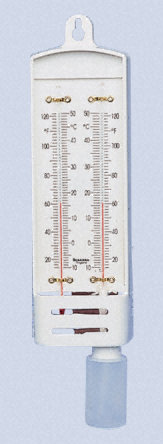This image features a double-sided outdoor thermometer with a white plastic backing. At the top, there is a plastic loop with a cutout center, designed to hook it to a wall. The thermometer includes two mercury-filled tubes side by side, each encased in their respective columns. At the top of each column, there are small gold circles connected by a gold bar. The scales on both sides measure temperatures in both Fahrenheit and Celsius, ranging from 120°F (outer scale) and 50°C (inner scale) at the top, down to lower numbers at the bottom. The thermometer also features two small slits near the bottom, which are described as resembling a small cylinder or bottle. The instrument is lying on a light blue background, and although it has some labels and logos at the top and bottom, they are not clearly legible in the image.